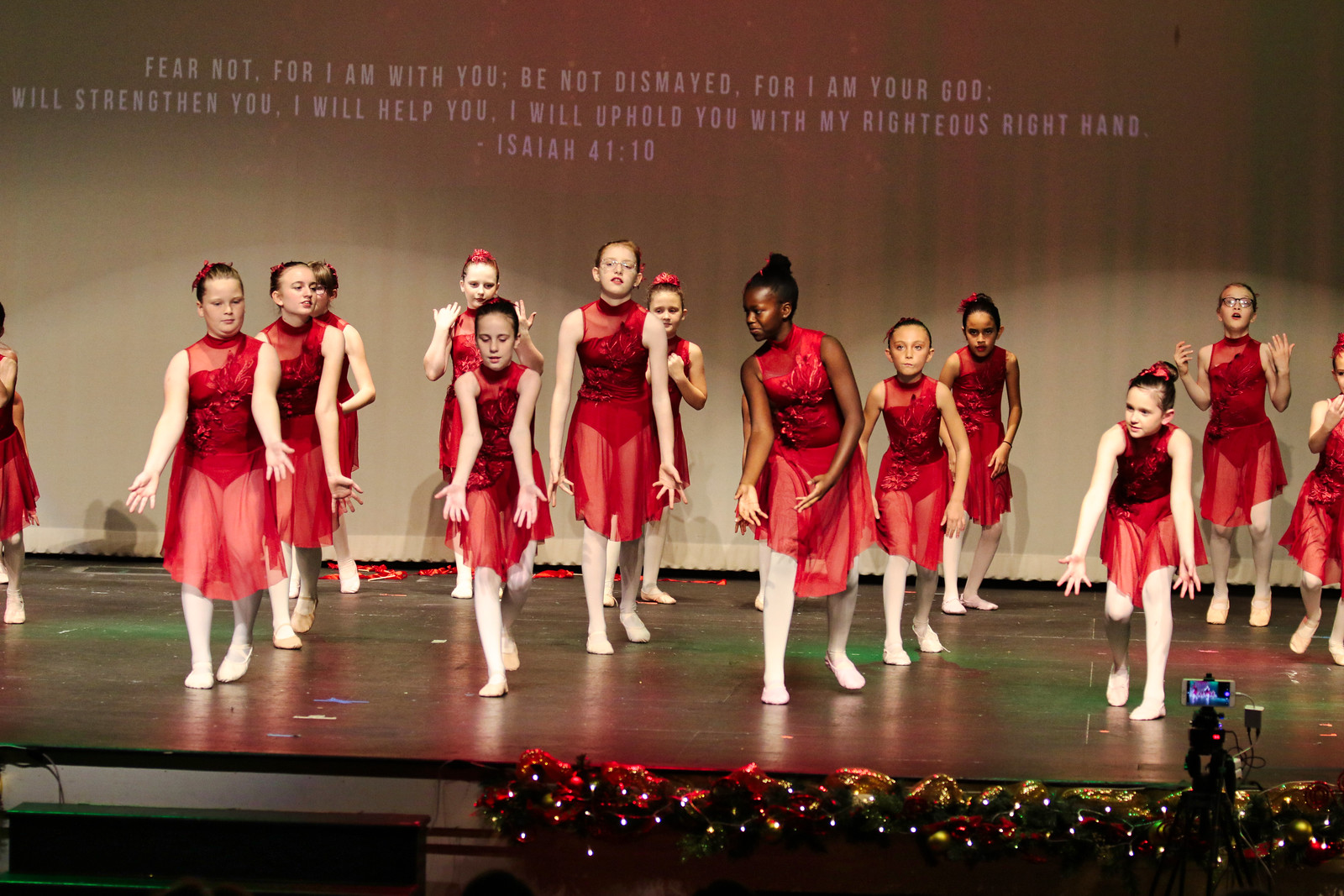The photograph captures a vibrant dance performance by a group of around 15 young girls arrayed on a stage. They are all dressed in eye-catching red bodysuits paired with gauzy, see-through red skirts, complemented by white tights and white dance shoes. The ensemble of largely Caucasian dancers, with a few dark-skinned girls positioned toward the center, strikes a variety of dynamic poses. Above them, a banner on the black stage wall displays a biblical verse, reading, "Fear not, for I am with you. Be not dismayed, for I am your God. I will strengthen you. I will help you. I will uphold you with my righteous right hand. Isaiah 41 10." This backdrop, in off-white text, frames the formal setting. At the foot of the stage, festive holiday lights add a touch of seasonal cheer, while a camera on a stand at the bottom right corner captures the performance. The background wall and floor feature natural colors, providing a subtle contrast to the dancers' vivid attire, making red the predominant color in this energetic scene.